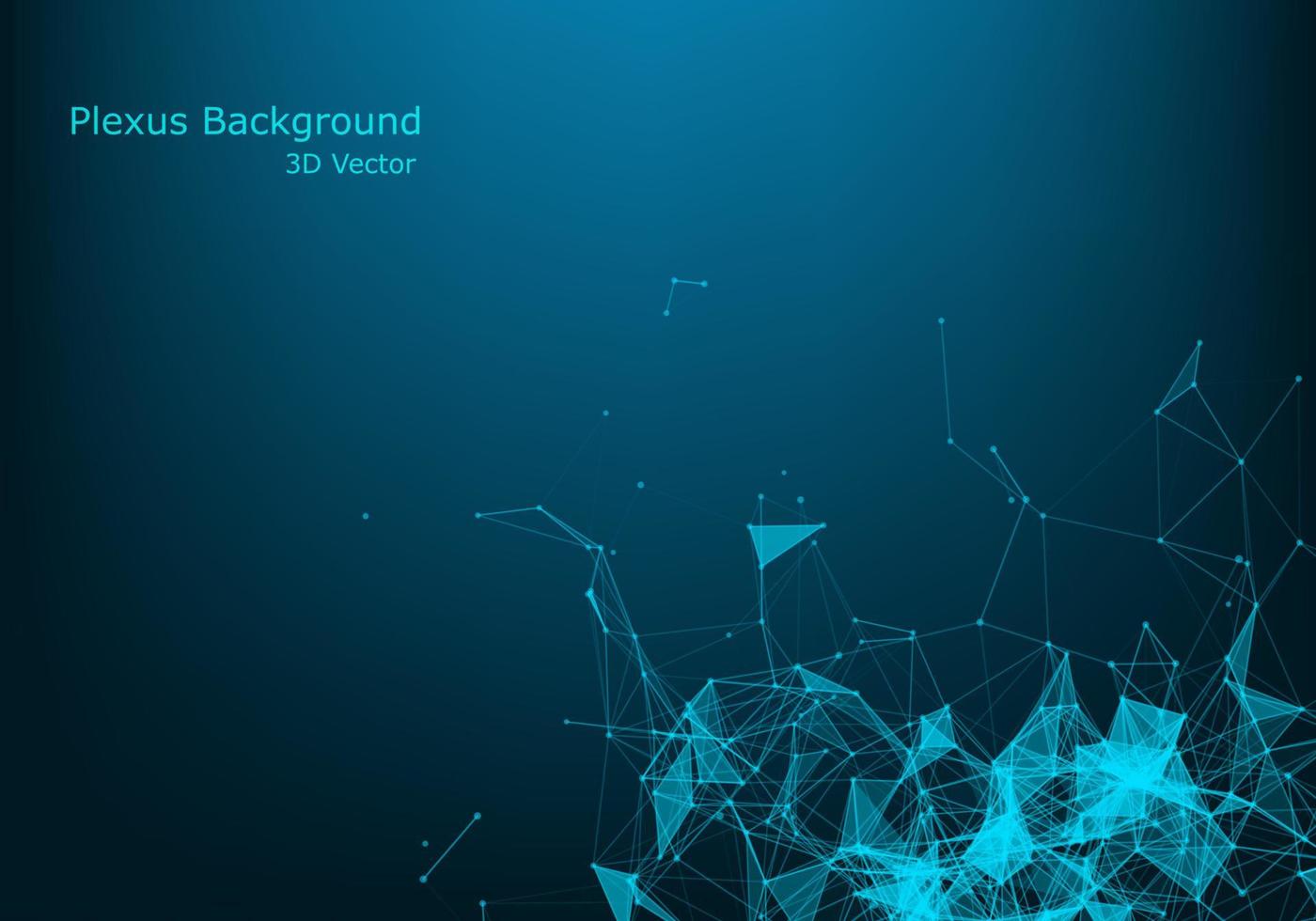This is a landscape-oriented image titled "Plexus Background 3D Vector" as indicated by teal text in the upper left-hand corner. The background transitions from a lighter blue at the top, suggesting a light source just above the image, to a darker, almost navy blue at the bottom. The lower right-hand corner is densely populated with an intricate network of white lines and dots, forming a series of interconnected triangles and diamonds. These shapes vary in color from fully white to light blue, adding dynamic color gradients to the image. Some shapes are filled, while others are merely outlined, contributing to a sense of depth and complexity. The geometric patterns resemble constellations, with a calculated arrangement that hints at underlying data points or mathematical principles, creating a visually compelling and intellectually stimulating design.